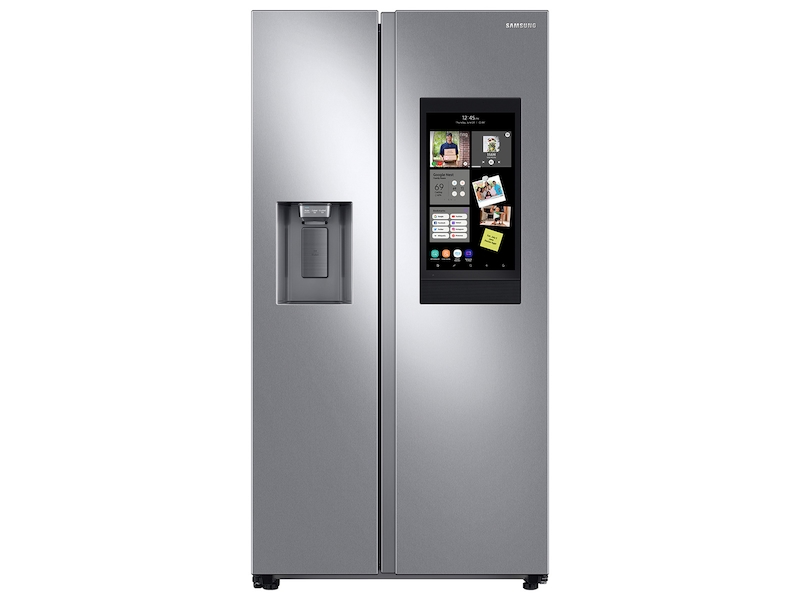The image showcases a sleek, Samsung stainless steel side-by-side smart refrigerator. The appliance features two doors that open from the center, with the freezer compartment on the left being slightly narrower than the refrigerator compartment on the right. A prominent Samsung logo is displayed in white lettering at the top right corner of the refrigerator door. The left door is equipped with an ice and water dispenser; users can place a glass beneath a silver lever to dispense ice. The right door features an expansive vertical black touchscreen display resembling a smartphone interface. This screen provides a multitude of smart features, including a clock, weather updates, music playback, grocery list creation, and the ability to view and manage the refrigerator's contents digitally. What sets this screen apart is its option to turn transparent, allowing users to see inside the refrigerator without opening the door. A slightly darker silver bar separates the two compartments, and black caster wheels at the bottom enable easy mobility. Overall, it is a modern, technologically advanced, and user-friendly household refrigerator.